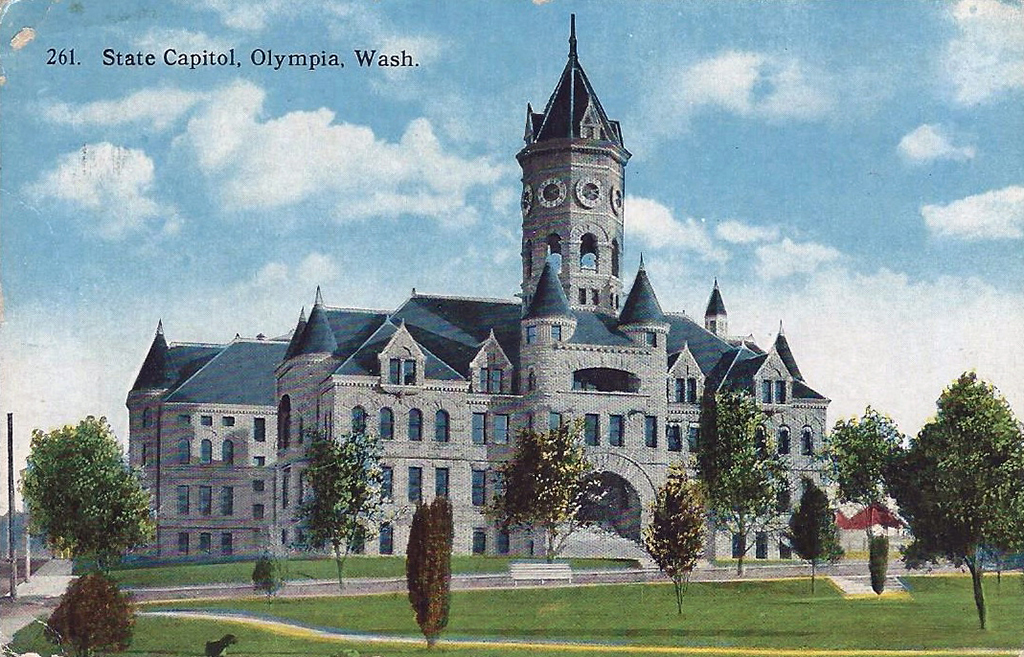The image appears to be an old, colorized illustration or a historically recreated photograph of a grand and imposing building labeled "261 State Capitol, Olympia, Washington" in the upper left corner. The building, made of gray brick and featuring a striking blue roof, is incredibly large and spans approximately four stories. Dominating its structure is a massive central tower adorned with clocks, capped by a blue top. The roof is adorned with numerous blue cone-like turrets.

The illustration is set in an outdoor environment with a vast green lawn in the forefront, dotted with eight different varieties of trees but no flowers. A walkway and benches are placed around the lawn, contributing to a park-like setting. The sky above is depicted as a vibrant blue with fluffy white clouds, enhancing the serene and majestic ambiance of the scene.